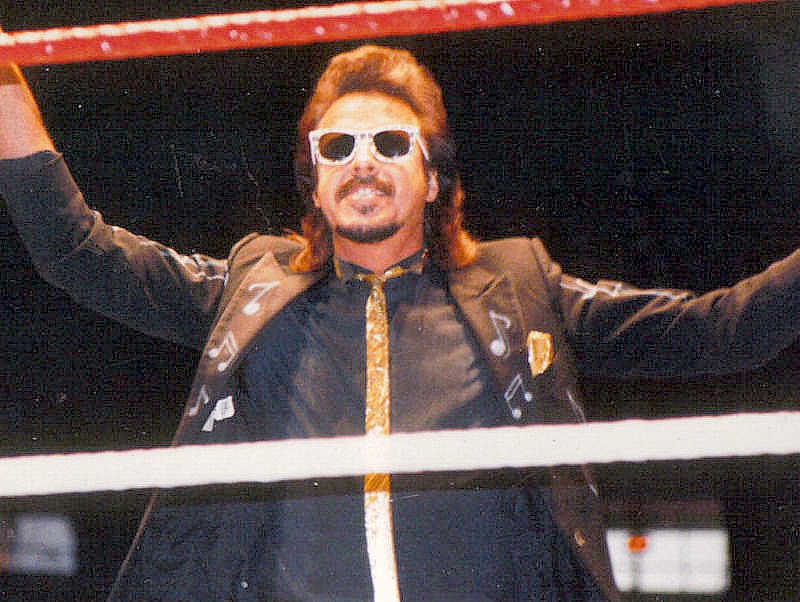The image depicts "The Mouth of the South" Jimmy Hart, a familiar figure from the former WWF, now known as WWE. He is positioned either entering or exiting a wrestling ring, as evidenced by the visible red and white ropes around him. Jimmy is dressed in a black blazer adorned with white music notes, over a black button-down shirt and a thin golden tie. Notably, he sports a gold handkerchief in his left jacket pocket. His long, poofy dark hair cascades to his shoulders, and he has a well-defined dark mustache and goatee. He wears sparkling black-framed sunglasses with white accents resembling diamonds. His arms are raised in a celebratory pose, and he has a congenial smile on his face. The background is predominantly dark, enhancing the brightness and clarity of his colorful outfit and joyous expression.